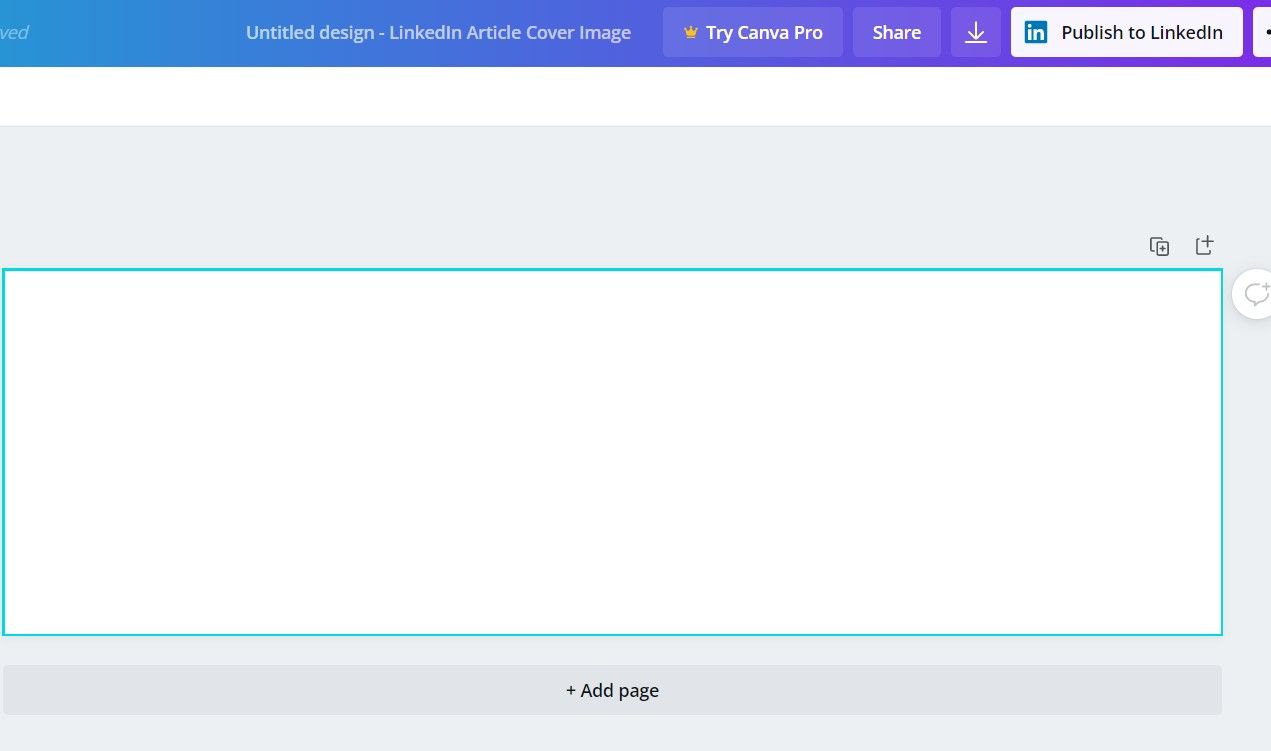The image depicts a product page for Canva Pro, showcasing a clean and minimalist design dominated by a white background, which constitutes approximately 90% of the photo. At the top of the page, a blue heading catches the eye with white text reading, "Untitled Design - LinkedIn Article Cover Image." Adjacent to this heading is a prominent rectangular button labeled "Try Canva Pro."

Next to the "Try Canva Pro" button is a smaller rectangular button offering a sharing option, and beside it, a smaller square button featuring an arrow pointing downward, signifying a download option. To the left of this download button, there is text reading "Publish To Link," which is encapsulated within a button format.

Beneath these headings lies a plain white heading, leading down to the main body of the webpage. The body section presents two primary options for adding content: a plus symbol indicating the ability to add new elements, and a chat symbol to the right, likely representing access to a chat box or support feature.

At the bottom of the page, there is an option to add a new page, marked by a plus symbol next to the "Add Page" text. This detailed layout highlights the functionality and user-friendly design of the Canva Pro product page.